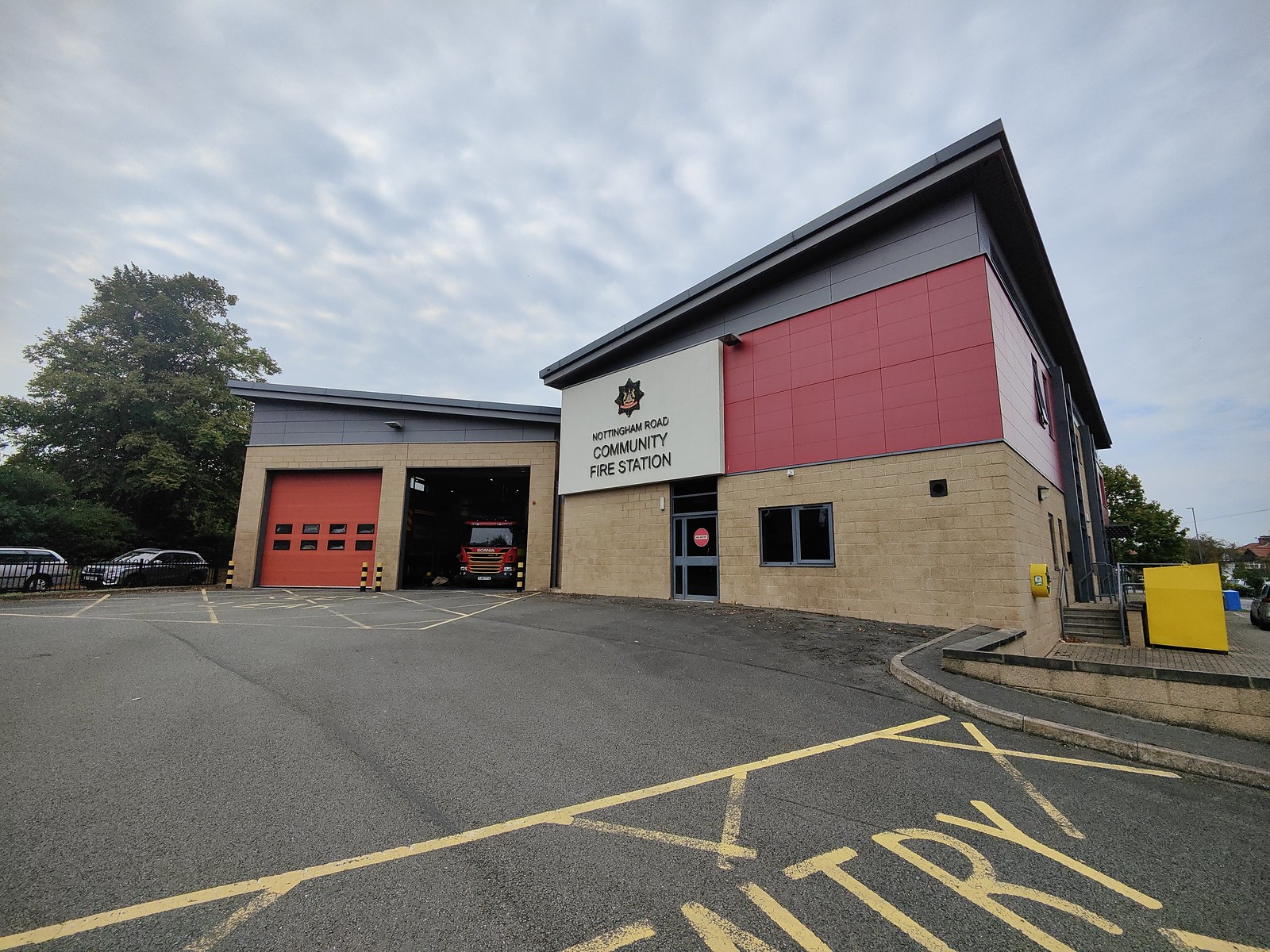The image depicts the exterior of the Nottingham Road Community Fire Station. On the left side of the station is a green tree near two garage doors; one door is red with eight windows arranged in two rows of four and is closed, while the other is open, revealing the front of a red fire truck inside. The building features a distinct tri-color scheme with light brown bricks on the lower level, red bricks in the middle, and a dark navy roofing. The tan brick part of the structure supports a large white sign bearing the fire station's name and a star-shaped logo above the entry door. This entry door has a metal frame with glass panels and is accompanied by a sizeable sliding window to its right. Additionally, there’s a brick wall segment and stairs leading up the building. In front of the station, the pavement features yellow markings with partial visibility of the word "entry," likely indicating traffic instructions. Various cars are parked outside amidst the surrounding scenery, with a backdrop of clear sky completing the composition.